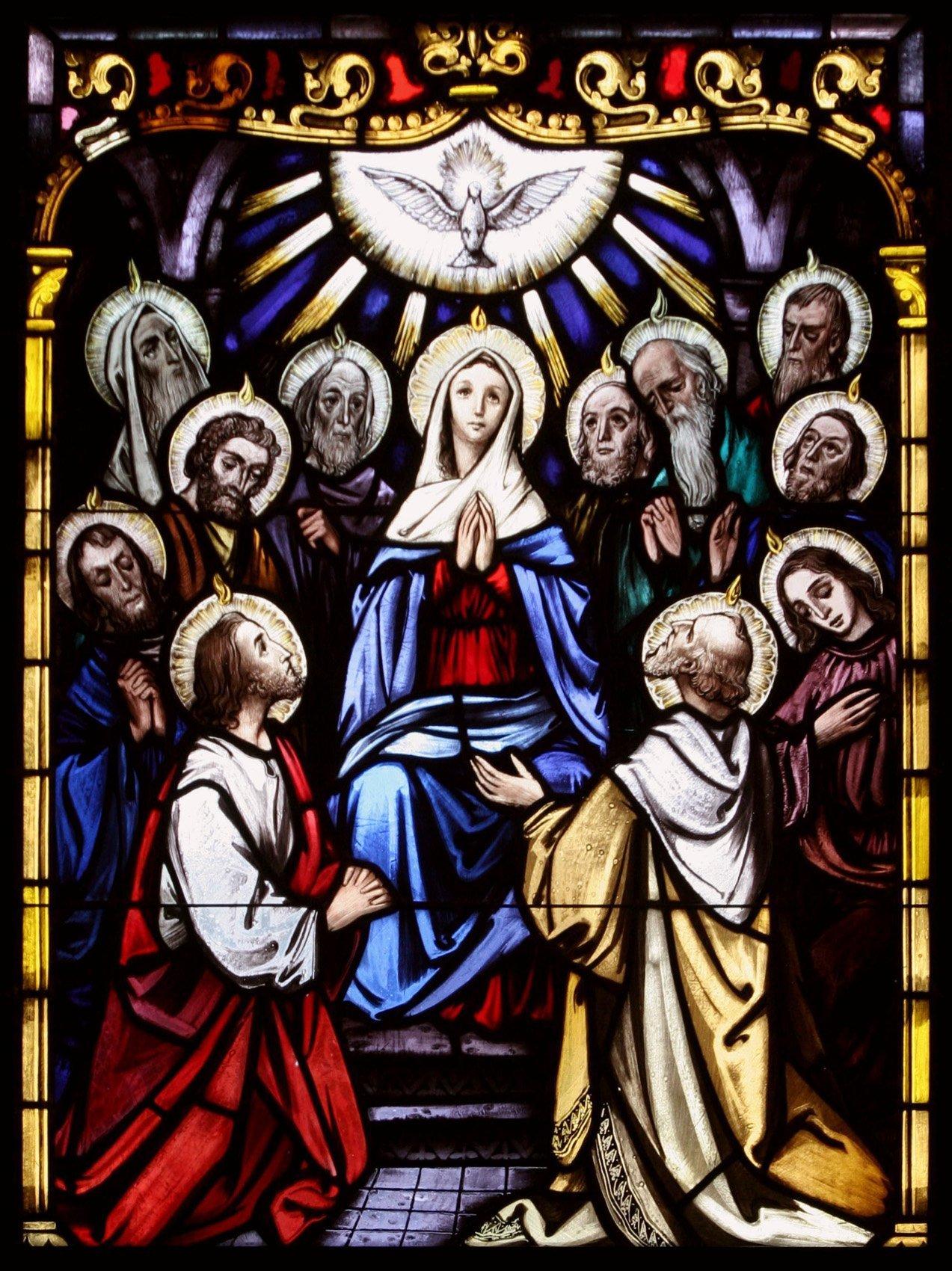This impressive painting is designed in the style of a stained-glass window, reminiscent of those found in grand Christian cathedrals. At its center, it features the figure of Mother Mary, draped in a green robe overlaid with blue, and a white cloth covering her head. Mary's hands are clasped in prayer as she looks upward with a serene expression. A halo encircles her head, and a brilliant sunbeam radiates from above, where a white dove with spread wings and its own halo is depicted. Surrounding Mary are eleven solemn saints, predominantly older men with beards, though one figure's gender is ambiguous. Each of the saints wears robes in a variety of vibrant colors, such as red, yellow, and green, and they all share the common feature of halos adorned with small wisps of flame. Arranged reverently around Mary, with some at her feet and others standing behind and beside her, they are depicted in postures of prayer and adoration, gazing either at Mary, the dove, or each other. The entire scene is encased in an ornate, golden frame, enhancing its rich, colorful, and devout imagery.